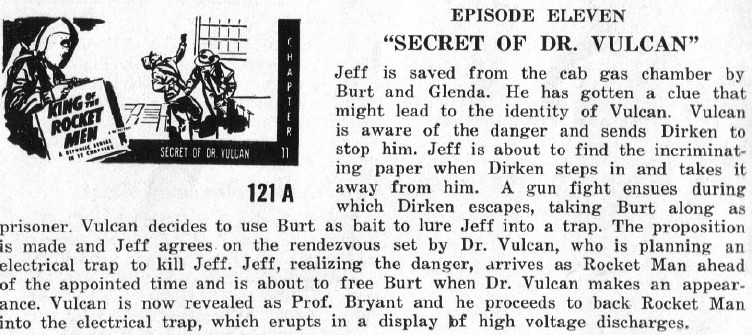The image is a detailed black-and-white illustration positioned at the top left corner of a page, depicting two men in the midst of a physical altercation. The accompanying text is an excerpt from "Episode 11, Secret of Dr. Vulcan," which tells a gripping story. Jeff is rescued from a dastardly cab gas chamber by his allies, Bert and Glenda. Armed with a crucial clue that might reveal Dr. Vulcan's true identity, Jeff becomes the target of Vulcan's henchman, Durkin. As Jeff is on the verge of discovering incriminating evidence, Durkin intervenes, seizes the paper, and a gunfight erupts. Durkin manages to escape, taking Bert as a prisoner. Dr. Vulcan plans to use Bert as bait to trap Jeff. Jeff agrees to the meeting set by Vulcan, but suspects an electrical trap lies in wait. Arriving ahead of schedule, Jeff attempts to free Bert, but Vulcan and the threat of high-voltage discharges loom large. The entire page, including the illustration and text, maintains a monochromatic aesthetic, lending a stark and intense atmosphere to the narrative.